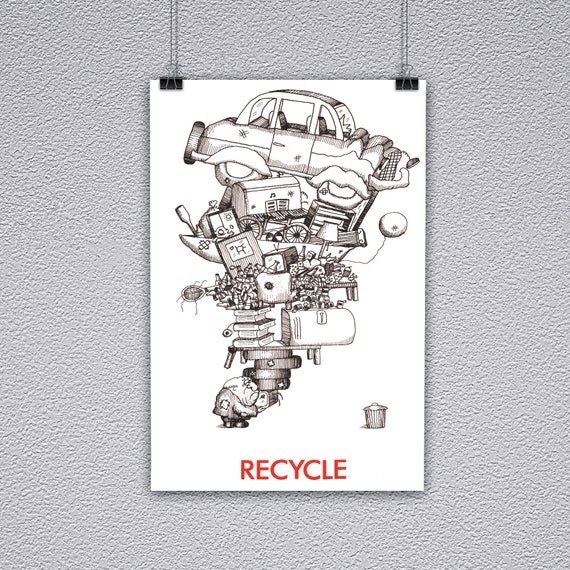The image features a black-and-white hand-drawn poster that is clipped and suspended from a textured light grey wall. The poster prominently displays the word "RECYCLE" in bold, red capital letters at the bottom center. To the left of this text, there is a small illustration of a garbage can. The main illustration depicts a small cartoon figure at the base, struggling to support an enormous, teetering pile of various objects arranged in ascending size. Starting from the top, the pile includes an old, two-door car, various tires that evoke the appearance of lips, an old bicycle, a television, bottles, books, a refrigerator, a boat filled with miscellaneous items, picture frames, a lampshade, a balloon, a mailbox, and a bookshelf. The drawing conveys an impactful message about the importance of recycling to prevent the accumulation of waste in landfills.